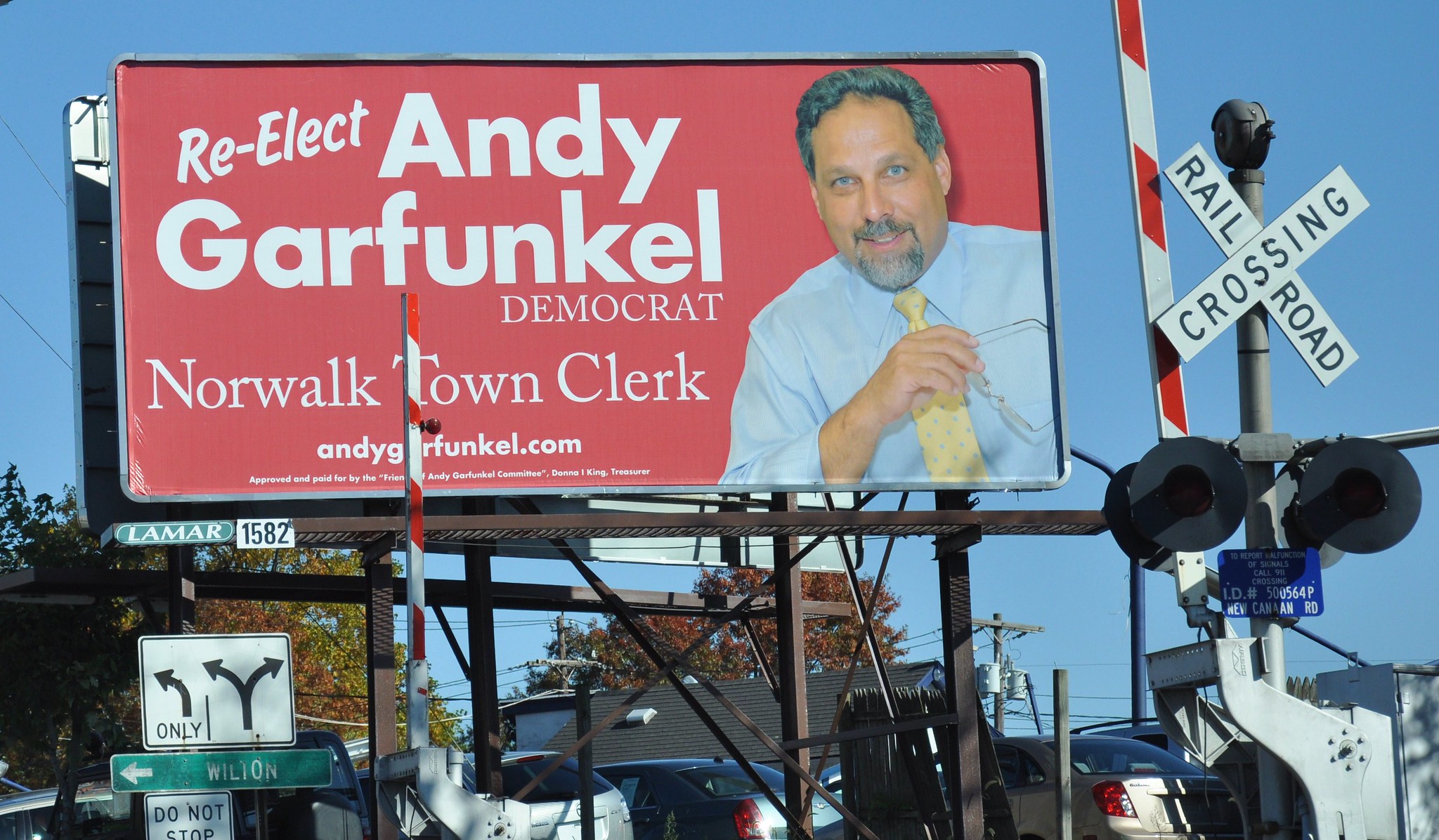This image is a horizontally oriented, close-up photograph of a billboard situated outdoors on a clear, cloudless day. The billboard features a red background with white text. Prominently displayed on the left side of the billboard is the message: "RE-ELECT Andy Garfunkel, Democrat, Norwalk Town Clerk," with "RE-ELECT" written diagonally across the upper left corner, and "Democrat" in all capital letters below Andy Garfunkel’s name. Near the bottom of the billboard, almost at the very edge, is the website "andygarfunkel.com" in lowercase letters. 

On the right side of the billboard is an image of Andy Garfunkel himself, depicted from the mid-chest up. He is a middle-aged to older gentleman with short gray hair, a neatly trimmed mustache, and a goatee. He has light tan, possibly slightly olive-colored skin, and blue eyes. He is dressed in a professional manner, wearing a light blue button-up shirt with a yellow tie, and he is gazing off with an engaging smile.

Adjacent to the right of the billboard is a railroad crossing sign, which includes a white cross with "RAILROAD" written on one diagonal bar and "CROSSING" on the other. The red and white gate arm is up, and beneath it, there are black railroad lights that are currently off. To the left of the billboard, there's a scene featuring fall foliage and various road signs. One white sign with black text directs traffic to turn left and right, a green sign pointing towards "Wilton," and a black and white "Do Not Stop" sign. Below the billboard, there are brown poles supporting it, and several cars are lined up behind, including a white car, a dark gray car, and a light gray car. In the background, buildings and electrical wires are visible, indicating the location might be a small or medium-sized town.